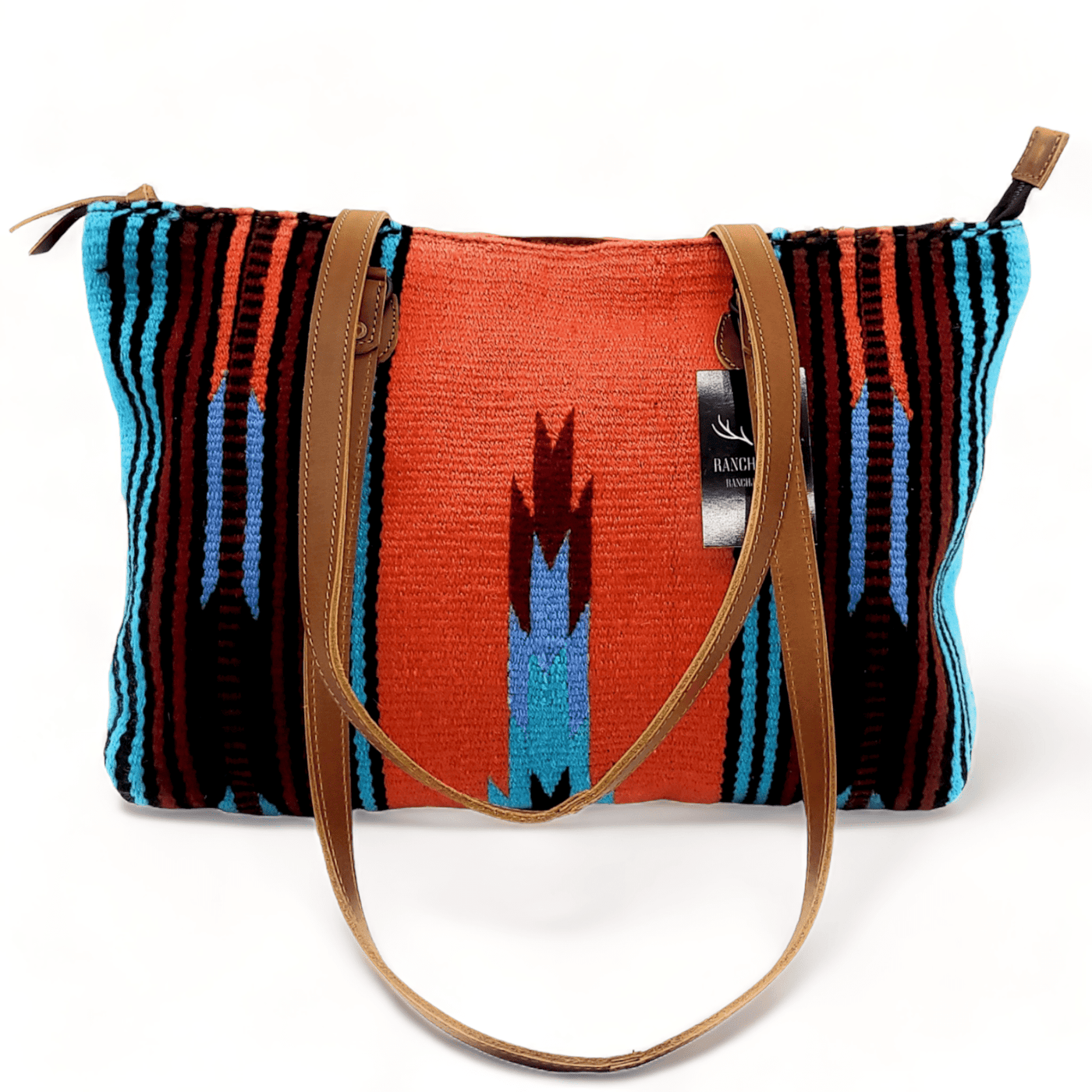This photograph features a handwoven purse with a rich, Native American-inspired pattern. The purse is crafted from a coarse woven yarn or thread material, providing a natural and tactile aesthetic. Its colors include a predominant central block of orange interspersed with a geometric column of teal blue and maroon. Flanking this central pattern are stripes in various hues, including teal, black, light blue, red, and additional orange accents, contributing to its vibrant, Navajo-like design.

The purse is equipped with two medium brown leather handles that are flopped over in the photographed position, enhancing its rustic look. Additionally, it sports a zipper at the top, capped with leather at the tip to cover the metal end, seamlessly blending functionality with style. The overall shape of the purse is rectangular, and it appears to be full rather than empty.

A small tag or logo is partially visible on the purse, bearing the word "ranch," suggesting a potential brand or design inspiration. The purse is set against a white background, emphasizing its intricate multicolored design and woven texture.